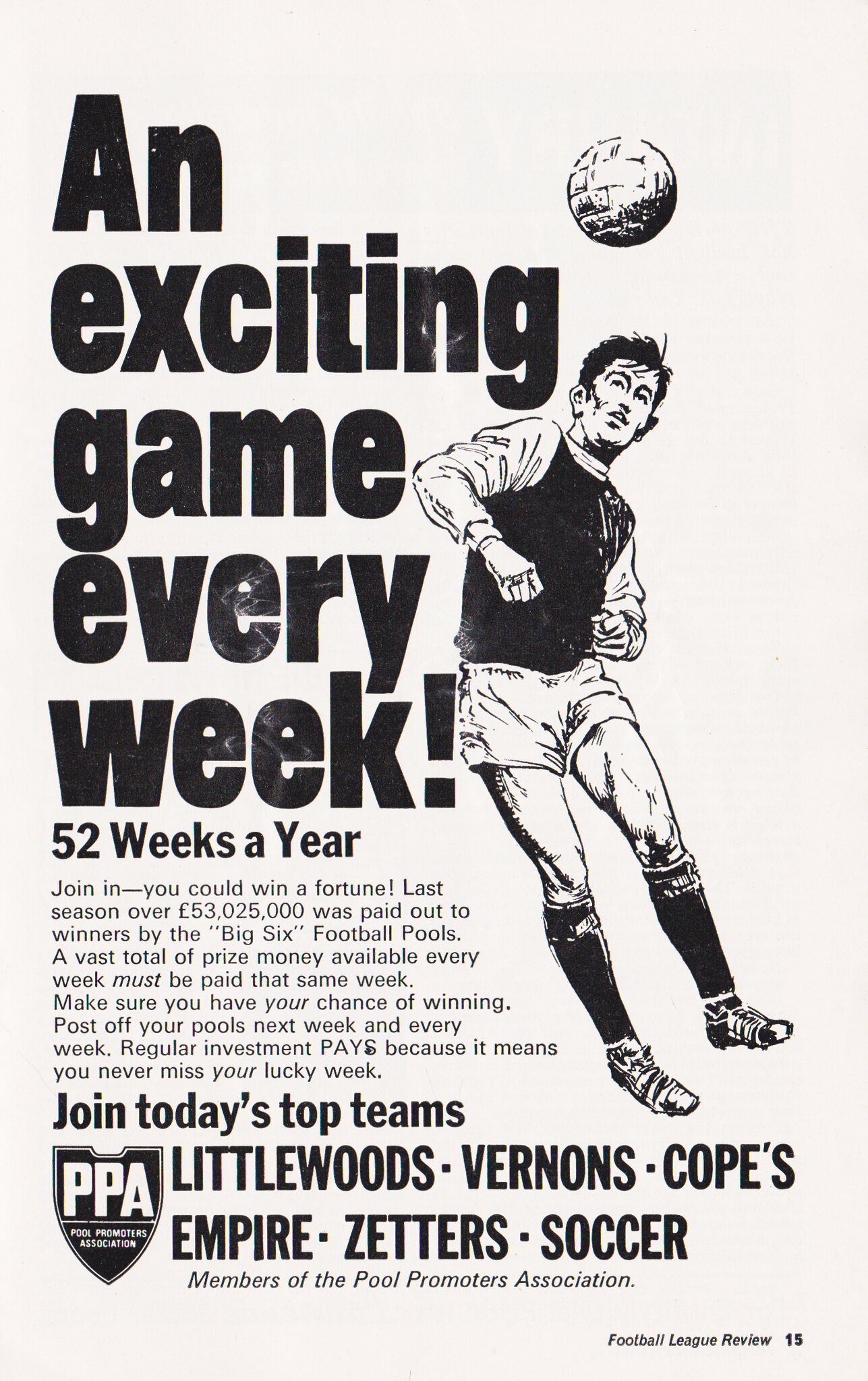This is a black-and-white advertisement featuring a photograph or drawing of a man in a soccer uniform, mid-jump, heading a soccer ball. Bold letters proclaim "An Exciting Game Every Week." Beneath this, the text reads "52 weeks a year. Join in. You could win a fortune." It highlights that last season over £53,025,000 was paid out to winners by the "Big Six" football pools. The ad emphasizes the substantial prize money available weekly that must be awarded within the same week, encouraging readers to ensure their participation by posting their pools every week. It mentions that regular investment ensures players never miss their lucky week. The ad concludes by inviting readers to join today’s top teams: Littlewoods, Vernons, Copes, Empires, Zetters, and Soccer, who are all members of the Pools Promoters Association. The text is set against a white background with black lettering, enhancing its straightforward, promotional message.